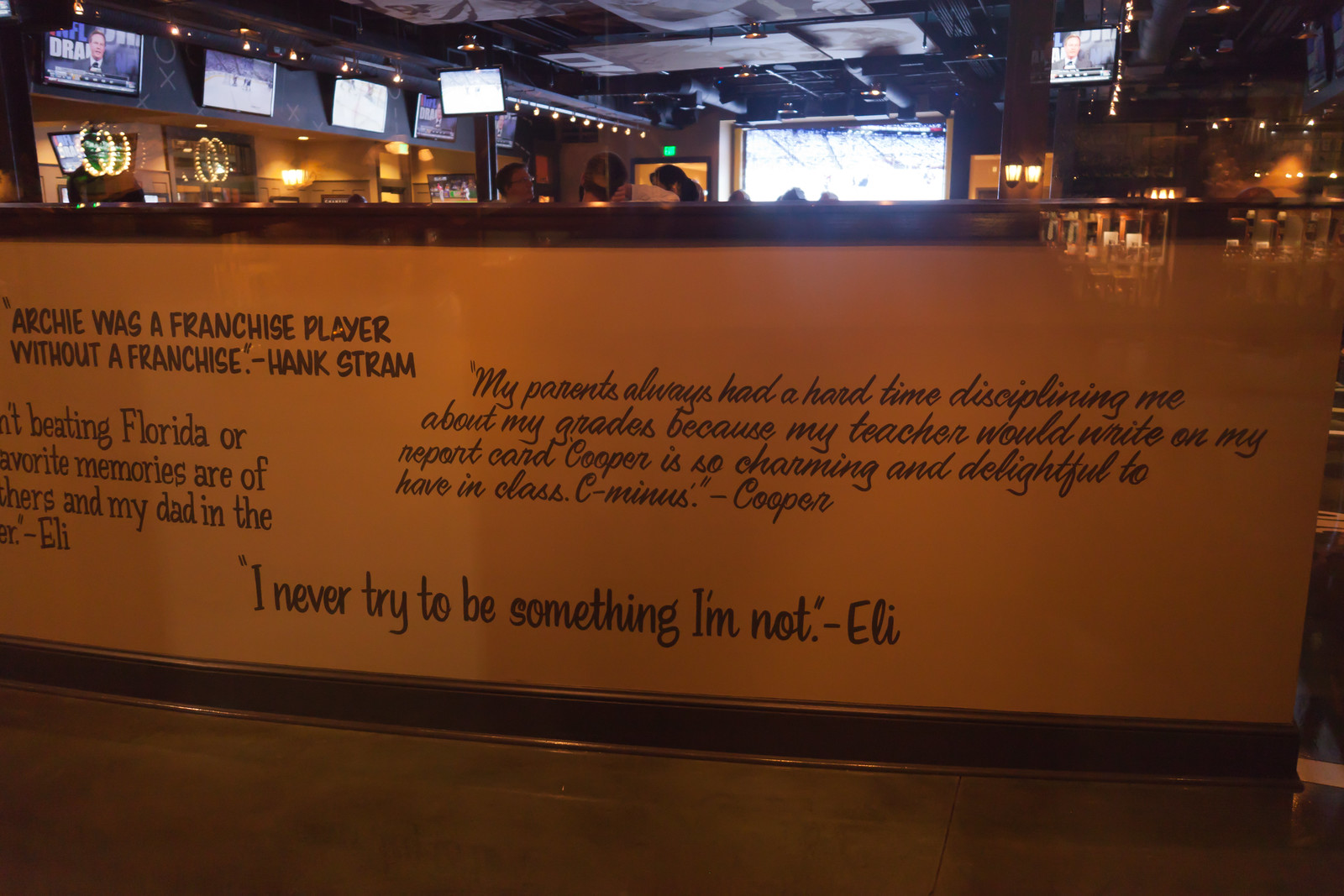This color photograph captures the interior of a bustling sports bar, focusing on a short, dark brown-bordered wall adorned with quotes from various famous personalities. Prominently displayed in cursive text, one of the main quotes reads, "I never tried to be something I'm not," signed by Eli. Above it, another quote amusingly notes, "My parents always had a hard time disciplining me about my grades because my teacher would write on my report card, Cooper is so charming and delightful to have in class, C minus," attributed to Cooper. On the left, partially visible, a quote reads, "Archie was a franchise player without a franchise," authored by Hank Stram. In the background, the top section of the image reveals several TV monitors affixed to the walls, broadcasting a mix of news and sporting events, including a hockey match and a scene with two men in tuxedos conversing. The photograph captures a lively atmosphere, with blue light streaming through an opening and glimpses of patrons' heads engaged in conversation over the top of the bar.